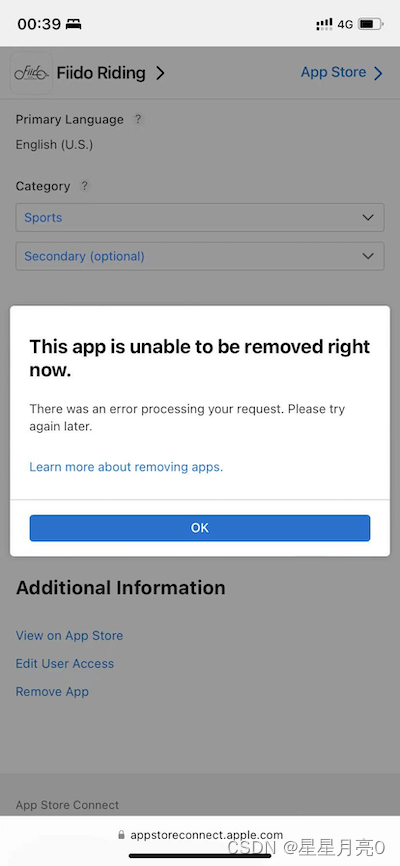A dialogue box appears on the screen, displaying a notification that reads "This app is unable to be removed right now" in bold. The user seemingly attempted to delete the app, but encountered an issue. Below the bold text, a message says "There was an error processing your request. Please try again later." Underneath this message, a blue link states "Learn more about this" with an "OK" button to close the dialogue box.

The dialogue box is white, and at the top of the screen, the time is displayed in military format as "03:09 hours." To the right side, there are indicators for battery level, 4G connectivity, and signal strength—grayed out due to the dialogue box overlay.

In the background, the app appears to be related to "Fido" with an emblem to the left of the text. On the top-right corner, there is another text in blue labeled "App Store." Below "Fido," on the left side, in a smaller bold font, the primary language is displayed as "English (US)" with a question mark icon for more information. Another label below reads "Category" with two dropdown boxes - the first labeled "Supports," and the second labeled "Optional," both with blue dropdown text.

At the bottom of the dialogue box, there is a section that says "Additional Information" in black text. Underneath, a blue text link reads "View on App Store," followed by "Edit User Access" and "Remove App." The very bottom of the dialogue box has a grey text labeled "App Store Contact."